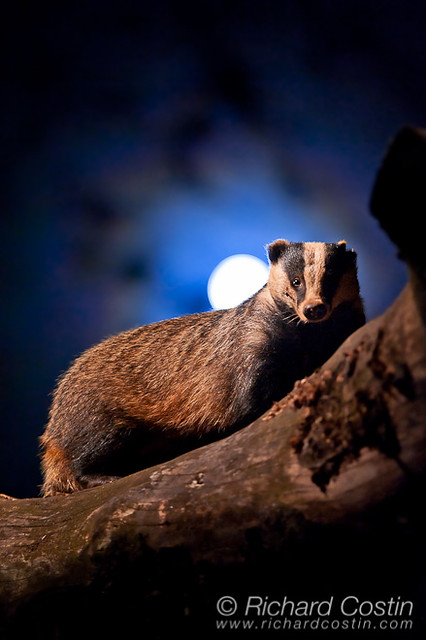In this captivating rectangular photograph by Richard Koston (www.richardkoston.com), a large adult badger is prominently featured resting on a substantial dried log that extends from the bottom left corner to the middle right side of the image. The badger, a rodent-like creature, boasts a distinctive tan-colored body with black fur on its front and striking black and white stripes adorning its head. Its tiny, rounded ears add to its robust yet charming appearance. The scene is bathed in moonlight, with the moon positioned just above the badger’s shoulders, framed against a backdrop of multiple branches and a deep blue night sky. The badger's gaze is fixed directly at the camera, giving a sense of fierce determination and toughness. The photograph is further certified with a copyright inscription at the bottom right corner that reads "Richard Koston, www.richardkoston.com."